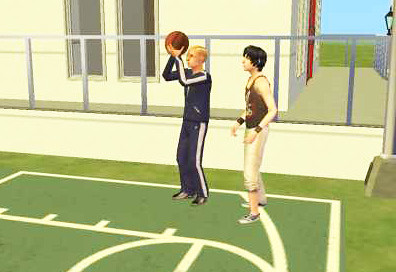The image is a computer-generated graphic of two boys playing basketball on a green basketball court near the three-point line, slightly to the right. The boy on the left, featuring blonde hair, wears a blue suit with white stripes along his arms and legs and appears to be facing left. The boy on the right, with dark hair, is dressed in a brown tank top and white pants rolled up to his calves. He also sports brown armbands and black and white sneakers, and he is holding a basketball over his head, poised to shoot. The court is surrounded by green grass, with distinct white lines marking the boundaries and key areas. In the background, there is a partial view of a white house with a silver metal railing and two visible windows.